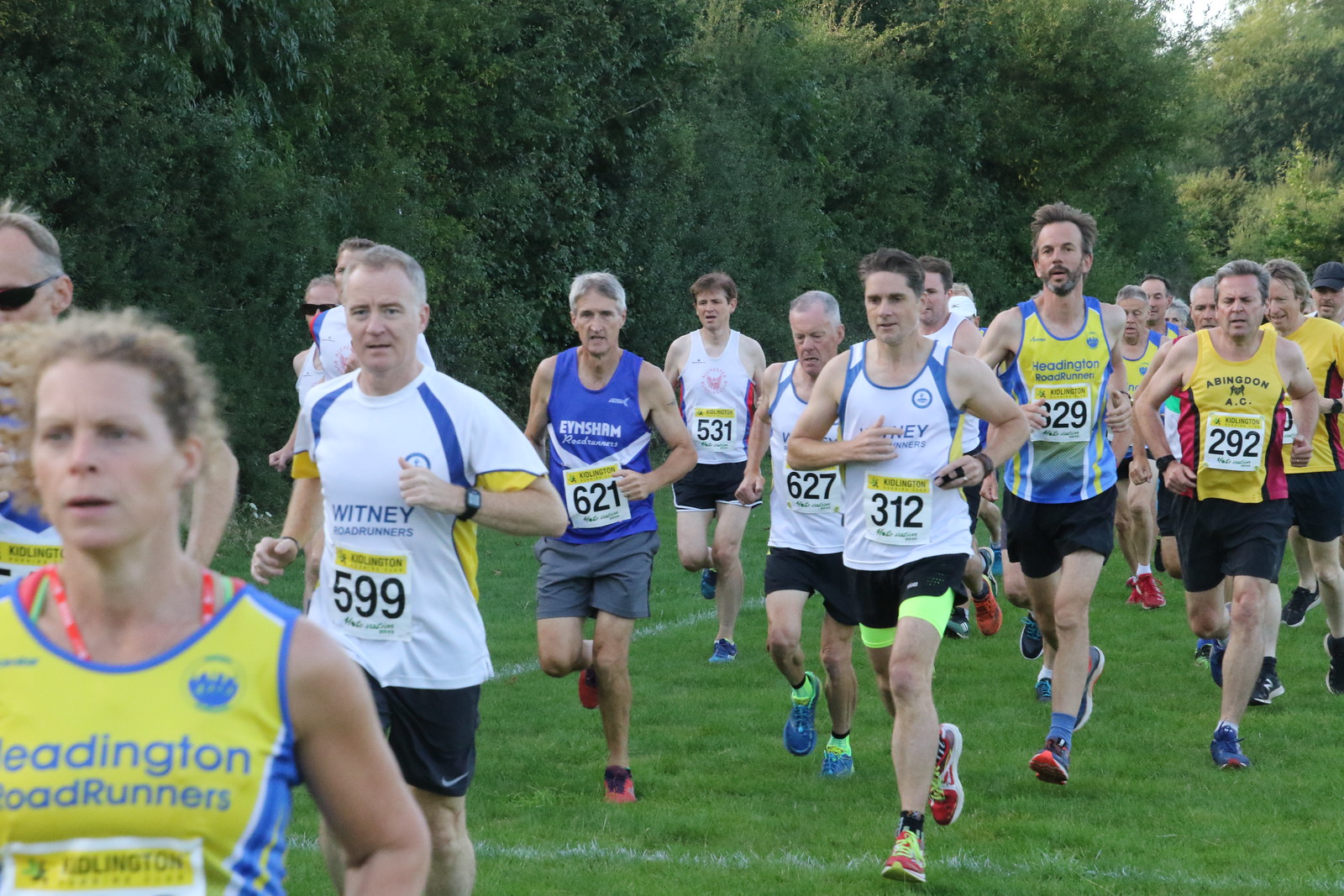The photograph captures an outdoor marathon on a partially cloudy day, featuring a large group of male runners from the Kidlington Road Runners club, distinguished by their numbered bibs—599, 621, 531, 627, 312, 329, and 292. The athletes are positioned towards the center, running towards the bottom left corner of the image across a green sports field marked with white chalk lines. In the middle and right portion of the group, runners are clad in yellow tank tops with black shorts and white tank tops with black shorts. Notably, a runner left of center is dressed in a blue tank top and gray shorts, while the leftmost individual sports a distinctive yellow and blue tank top with their race number obscured. The background displays dense bushes with a bit of visible sky, suggesting the race is taking place in a serene outdoor setting.